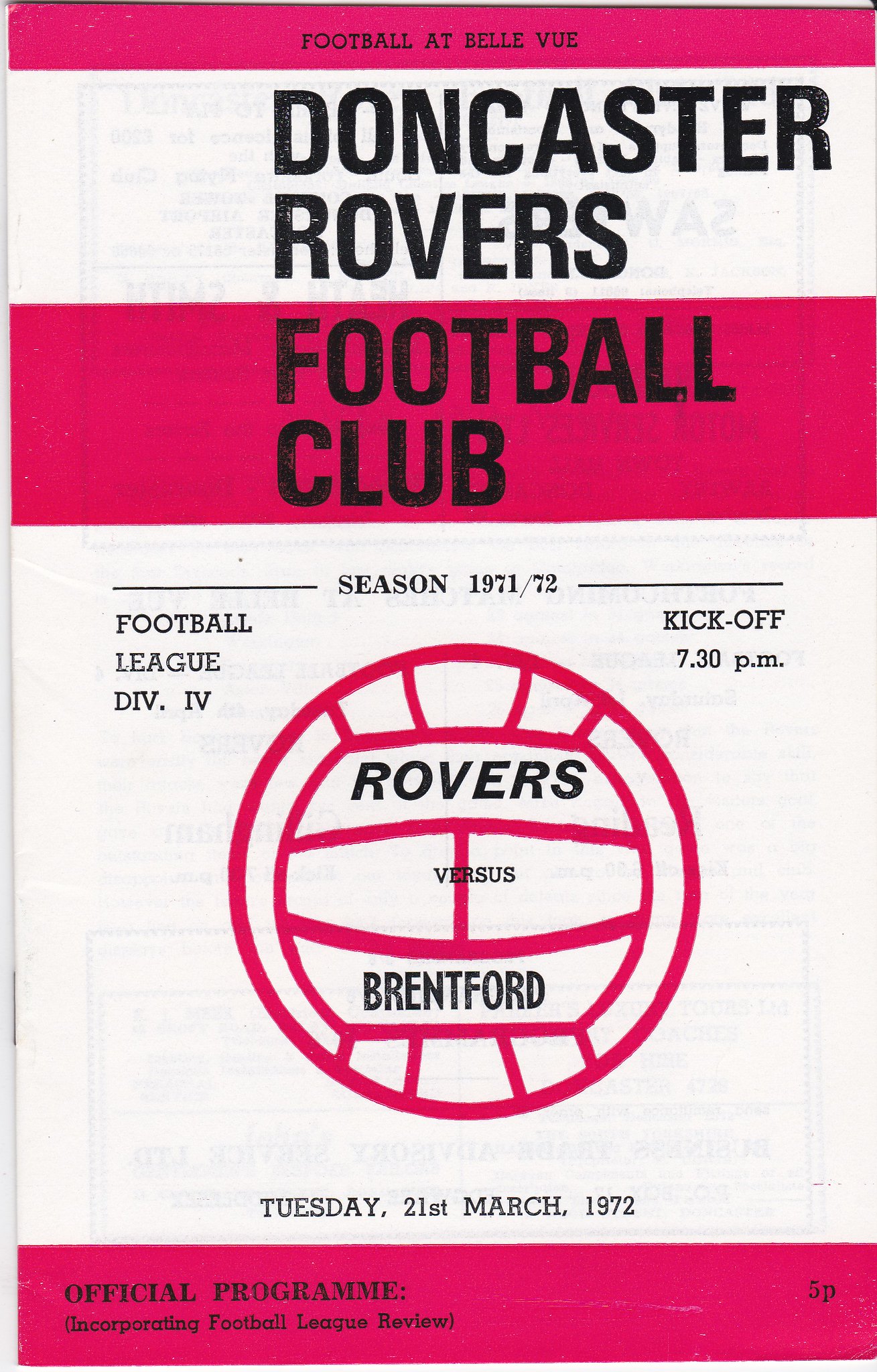This image presents the front cover of an official soccer program for a match at Bellevue. The cover is designed in black print with red spot ink on a predominantly white background. At the very top, in black lettering, it reads "FOOTBALL AT BELLEVUE." Directly beneath this, also in black, are the words "DONCASTER ROVERS." Below this title, a wider dark pink horizontal band displays "FOOTBALL CLUB" in bold black letters. 

The central part of the cover is largely white, featuring a prominent line drawing of a soccer ball in pink. Inside the ball, the text "ROVERS" appears prominently in black, followed by "versus" in smaller letters, then "BRENTFORD" in slightly larger letters. To the left of the soccer ball image, in black type, it reads "FOOTBALL LEAGUE DIV. IV," while to the right, it states "KICK-OFF 7:30 PM."

Above the soccer ball, the cover notes "Season 1971-72" in small black lettering. Below the ball, "Tuesday, 21st March 1972" is clearly printed. The bottom of the poster is marked by a dark pink rectangle stretching across the width, bearing the black text "OFFICIAL PROGRAM" priced at five pence and noting that it incorporates the "Football League Review."